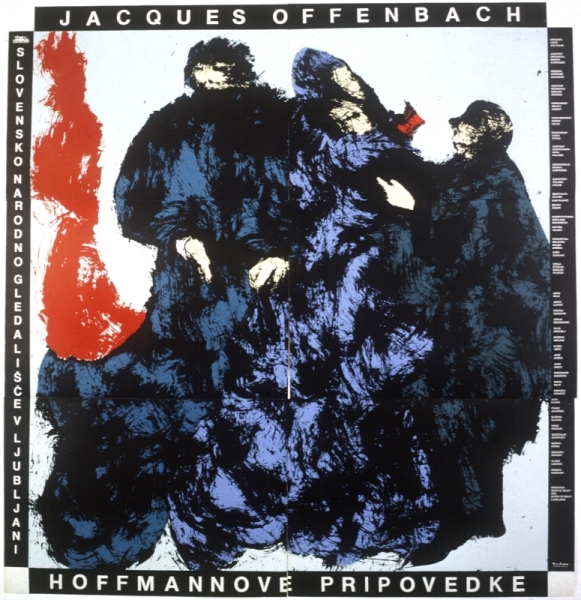This square image appears to be an album cover or an art piece featuring a central abstract scene. The top border has a black rectangle with "JACQUES OFFENBACH" in bold, white, capital letters. A vertical black rectangle on the left reads "SLOVENSKO NARODNO GLADALIŠTE V LJUBLJANI" in white, capital letters. The bottom border contains a black rectangle with the text "HOFMANOV PRIPOVEDKE," also in white, capital letters. The right side features a black vertical rectangle with very tiny, unreadable white font.

In the center of the image is an abstract painting with a white background. It showcases several figures adorned in large blue and light purple cloaks, with their faces and hands barely visible as white shapes. The figures' expressions are indistinct, and their forms blend with an adjacent area of red paint that splatters vertically from the upper left corner to the middle left edge. The overall composition exudes a mysterious, abstract aesthetic.